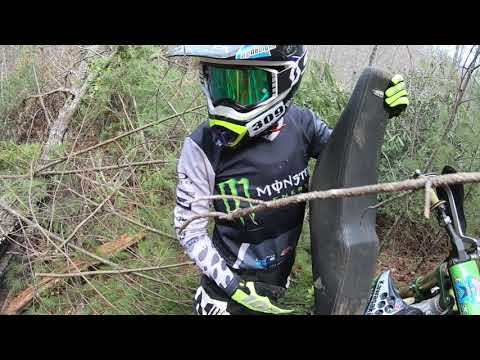In a dense, wooded area with limbs and trees forming the backdrop, a motocross rider stands prominently in the scene. The individual's face is completely obscured by a helmet bearing the number 309 and a face mask. The helmet features a striking green visor. They are dressed in specialized dirt biking attire, which includes a long-sleeved shirt emblazoned with the Monster Energy drink logo, featuring a dark blue torso with a dripping green 'M' and white sleeves adorned with various designs. Yellow gloves cover their hands as the person holds up the tipped motorbike, gripping both the handlebars and the seat, which exposes parts of the black motorbike. There are some logos on the shirt's sleeves, though their details are unclear. The sky is barely visible, peeking through the thick foliage, reinforcing the sense of seclusion in this rugged outdoor setting.